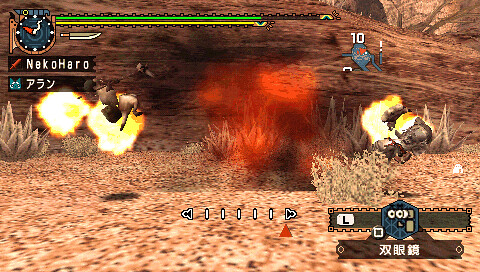The image is a detailed depiction of a video game screenshot. In the upper left-hand corner, the player's name "Neko Haro" is displayed, accompanied by a health bar in green and an energy bar in yellow, which is slightly shorter. Beneath Neko Haro's name, a little green fox and Japanese kanji are visible. On the bottom right-hand side, there are Chinese characters, along with an orange and black film reel-like icon with a letter L behind it, and a pentagon with a pair of eyes and additional Japanese kanji below it.

The main scene showcases a battle in a desert environment with dark orange, sandy terrain. The ground is dotted with six plants in the background and one green plant in the foreground. The combat involves two metal robot characters amidst an explosion, with one robot surrounded by two explosion animations and the other by one. Red fireballs are seen to the right and more fireballs in the center of the scene. A mini-map is located in the upper right-hand corner, featuring the number 10.